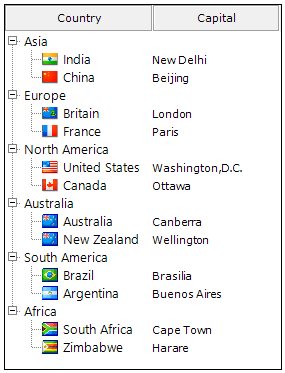The image displays a structured list segmented into blocks for "Country" and "Capital," each outlined with a thin dark gray border to distinguish them. The titles "Country" and "Capital" are emphatically displayed in bold black font, both starting with capitalized 'C'. On the far left, plus and minus symbols indicate that each category can be expanded or collapsed for detailed viewing. The list of countries and their respective capitals is shown in an expanded format.

At the top of the list, the category "Asia" is shown with sub-entries for 'India' and 'China.' Adjacent to each country name, the capitals are listed as 'New Delhi' for India and 'Beijing' for China. Directly below, the category "Europe" appears with sub-entries for 'Britain' and 'France.' Their capitals are indicated as 'London' for Britain and 'Paris' for France. The clean and organized layout provides a clear and concise reference for the countries and their capitals within the specified regions.